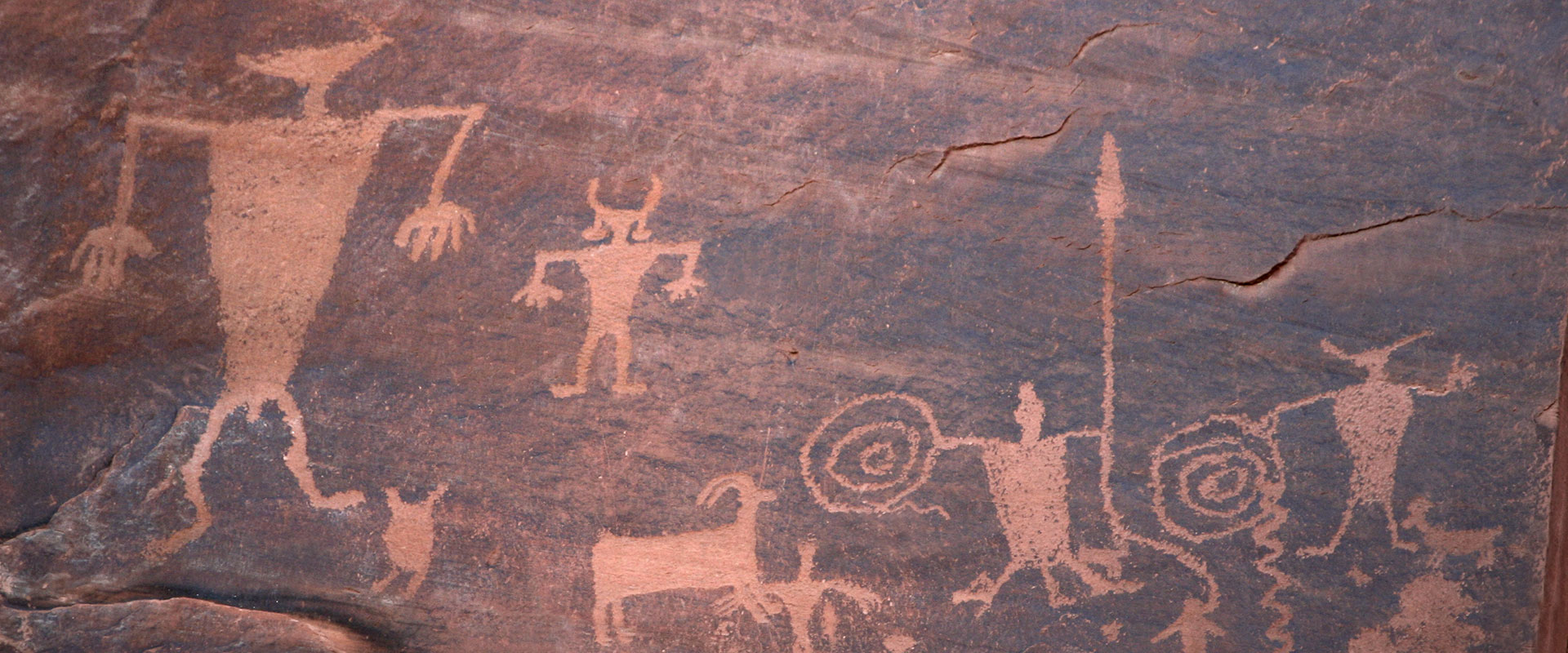This photograph captures an ancient cave painting etched into the soot-covered surface of a worn, gray stone wall inside a cave. The detailed art, predominantly in a natural tan color contrasted against the blackened rock, depicts a variety of human and animal figures. On the left side, the largest humanoid figure with a triangular head stands prominently, showcasing detailed limbs and fingers. Nearby, a smaller horned figure appears, holding a rope and a spear, while a goat-like animal is seen below it. To the right, an intricate series of circles resembling targets accompanies a turtle-like shape, which seems to clutch a stick. Additionally, the composition includes another horned humanoid figure and a creature resembling a dog. The rock shows visible signs of wear with cracks and an overall weathered texture, emphasizing the ancient and historical significance of the artwork.